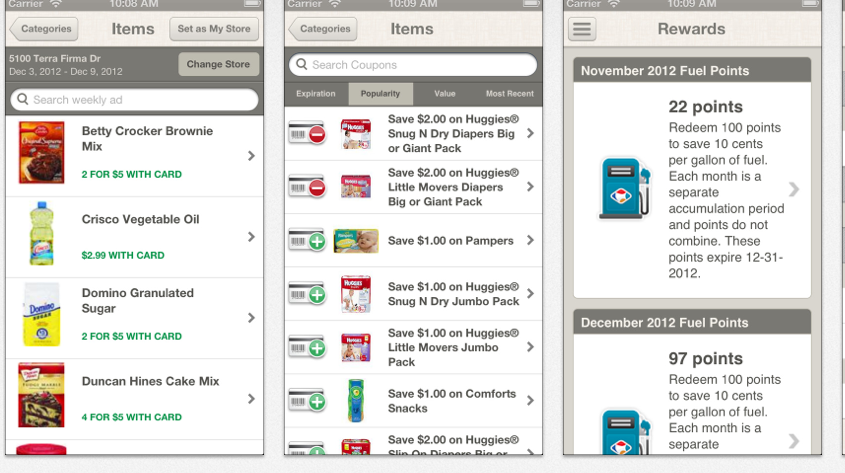This collage photo showcases three different mobile shopping app pages, each providing distinct features for a seamless shopping experience.

On the left, the image captures the "Items" category page. At the top, "Items" is prominently displayed in bold, gray font, centered. To the left of "Items," an arrow points left with the label "Categories" in small gray letters inside, suggesting a navigation option. On the right, there's a button labeled "Set as My Store." Below this, a gray box displays the store's address on the top left, accompanied by a "Change Store" button on the top right. The gray box also features a search bar with the placeholder text "Search Weekly Ad." Further down, a vertical list of products is visible.

The middle screenshot also depicts the "Items" page. Directly below the title "Items," a search bar is featured, allowing users to "Search Coupons." Below this bar, various categories are displayed horizontally: Expiration, Popularity, Value, Most Recent, with "Popularity" currently selected. A vertical list of available coupons follows.

On the right, the screen is focused on the "Rewards" tab. The word "Rewards" is centered at the top, followed by various offers aimed at earning fuel points, enhancing the user's shopping and savings experience.